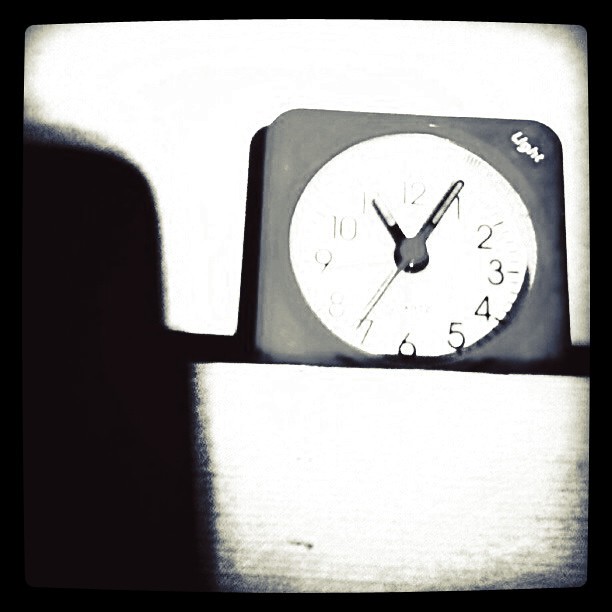This black-and-white photograph captures an old-fashioned, somewhat blurry and overexposed image of an analog clock, likely an alarm clock, with a distinctive square gray frame and a round face. The clock is positioned directly facing the viewer and displays the time as 5 minutes after 11. The numerals from 2 to 6 are clearly visible, while those from 8 to 12 are faded, possibly due to light exposure. The minute and hour hands are accompanied by a slender sweep second hand. The clock's hands and numerals seem to have a reflective material, designed to glow in the dark. The upper right corner of the clock bears a faint company logo starting with the letter 'U'. Shadows cast around the clock and a white wall in the background emphasize the photograph's vintage feel.